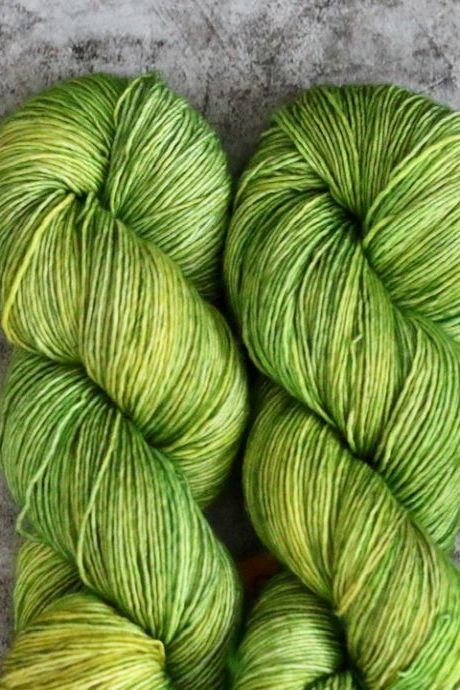This close-up photograph captures two skeins of lime green yarn intertwined in tight twists, resembling a braided infinity shape. The yarn showcases variegated hues, transitioning from lime green to shades of pale yellow, with some strands slightly unraveled yet mostly tucked neatly together. These yarns, appearing soft and ideal for knitting, rest side by side on a marbled surface featuring black, gray, and white markings. The image does not reveal the full length of the yarn as it is cut off at the bottom, emphasizing the intricate and repetitive pattern of the twist.